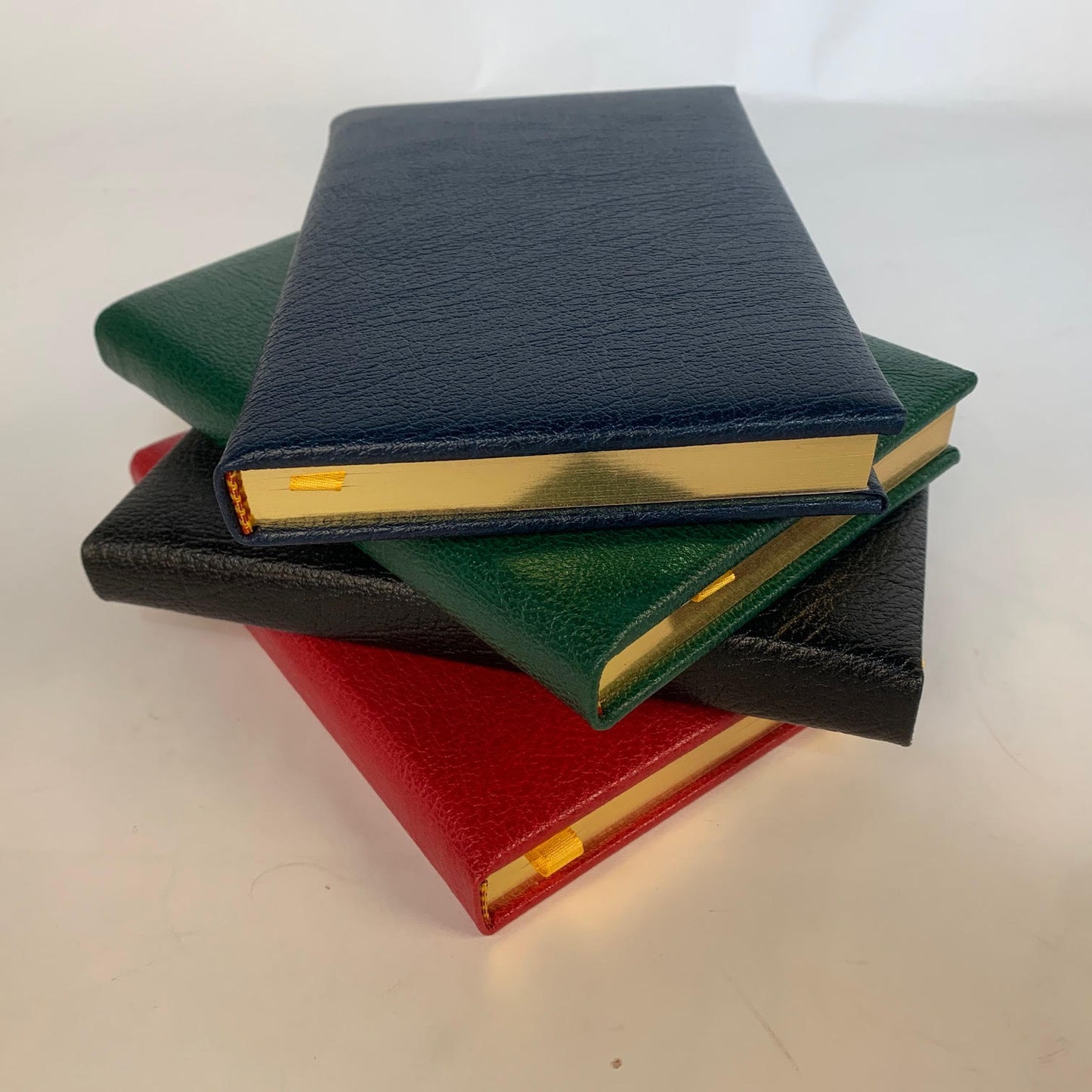This image features a stack of four leather-bound books arranged haphazardly on a tan background that resembles a cream-colored table. Each book is closed and hardcover with shiny gold-edged pages and yellow bookmarks tucked inside. The books are placed at different angles, creating an interesting visual effect. Starting from the bottom, the first book is red, angled with the top pointing toward the upper left corner and the bottom toward the lower right. Above it is a black book, tilted with the top facing the left middle and the bottom towards the right middle. The third book in the stack is green, positioned with its top end towards the upper left corner and the bottom end towards the right middle. The topmost book is blue, lying flat with the top end facing the upper middle of the picture and the bottom end directed straight toward the viewer.